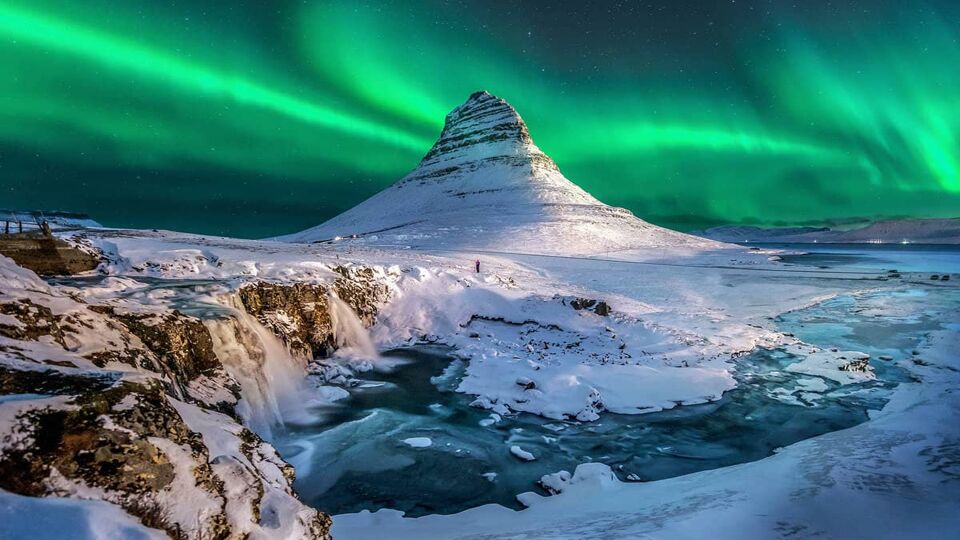The photograph is a high-quality, vibrant outdoor scene in Alaska, showcasing a cold, snowy landscape. In the background stands a uniquely shaped, pointed, possibly volcanic mountain blanketed in snow. The foreground displays a mix of snow-covered boulders and flowing deep blue water. This water cascades off a small cliff into a larger pool, which then transforms into a river heading towards the sea.

Amidst these elements, patches of broken ice reveal the water beneath, and on the right side, additional water is visible. Dominating the upper part of the image is the night sky, glowing with brilliant shades of green and blue from the northern lights. These lights create a stunning, curtain-like effect, adding a striking, almost surreal quality to the snowy and icy scene. There are no signs of human life or writing on the photograph, emphasizing the pristine and untouched beauty of this Alaskan wilderness.